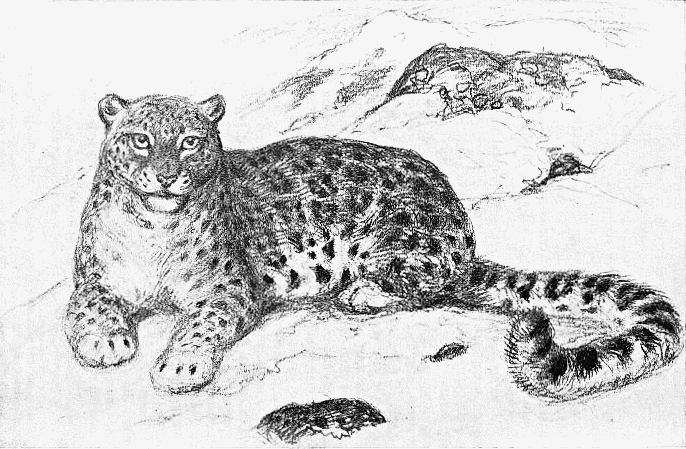The image is a detailed black-and-white drawing of a large spotted cat, likely a leopard. The animal is lying on the ground, with its two front paws extended forward and its body curled up in the back. Its long tail curves to the left, with the tip facing towards its head. The leopard's head is raised as if it's gazing into the distance, giving an impression of alertness. The cat is positioned on the left side of the picture, with its head and front paws facing the viewer, and its tail extending towards the right. The background features a contrast of dark rocky terrain, perhaps suggesting a mountainous or snowy environment. The scene depicts the cat in a natural habitat, with subtle details like its white chest, small ears, and piercing eyes enhancing the lifelike quality of the drawing.